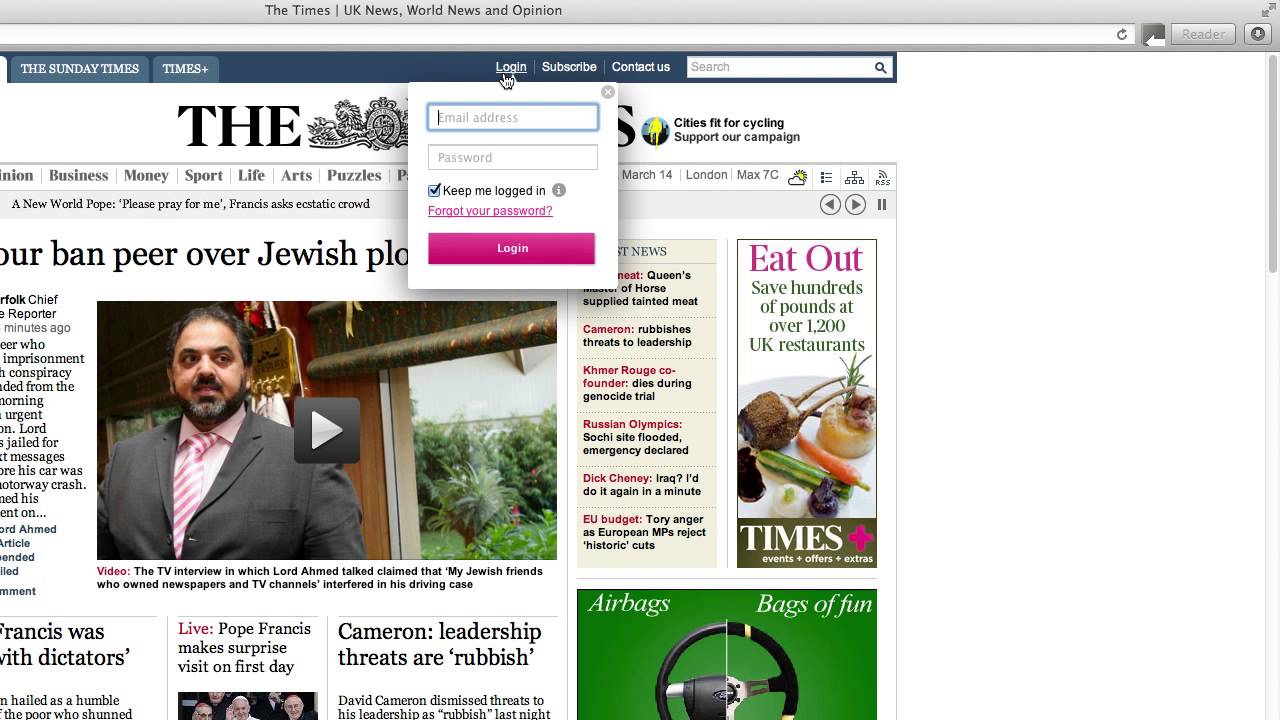A detailed caption for the described image:

The image depicts a webpage from "The Sunday Times," prominently featuring its recognizable newspaper icon at the top. The login screen partially overlays the main content, including fields for an email address and a password, alongside a "Keep Me Logged In" checkbox marked by a pink icon. The top-left corner identifies the site as "The Sunday Times" and includes the "Times Plus" label. The navigation bar lists sections such as "UK News," "World News," and "Opinions." A headline reads, "Our Ban Pier Over Jewish...", although the complete text is obscured. Adjacent to it is an image of a man in a grey suit, pink collared shirt, and pink tie, sporting a full beard. The caption for this image references a TV interview with Lord Ahmed, alleging interference by his Jewish friends who own media outlets in his driving case. Other headlines are visible, including, "Live: Pope Francis Makes Surprise Visit on First Day." The page is a blend of multiple colors, with an advertisement featuring a green background and black steering wheel. Most headlines are presented in black on a white backdrop.